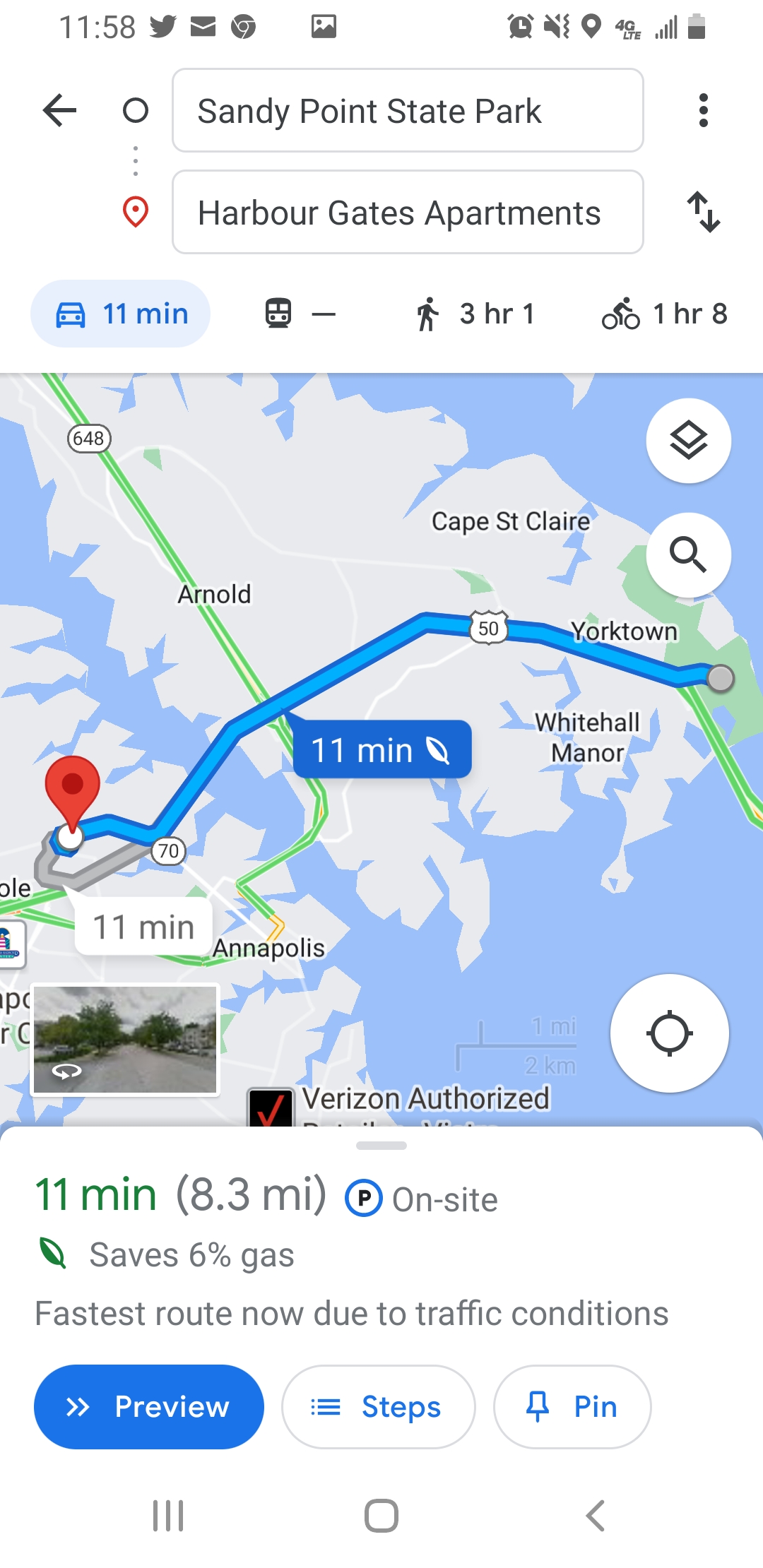This is a detailed screenshot of a Google Maps navigation screen on a mobile phone. The phone's top status bar displays typical icons such as app notifications, battery level, and signal strength. The screenshot maps a route from Sandy Point State Park to Harbor Gates Apartments. According to the map, traveling by car will take 11 minutes. There are no public transportation options available. Walking to the destination is estimated to take three hours and one minute, and cycling will take approximately one hour and eight minutes. The navigation is currently set to car mode. In the map layout, Sandy Point State Park is located on the right-hand side of the screen, and the route to Harbor Gates Apartments proceeds westward.